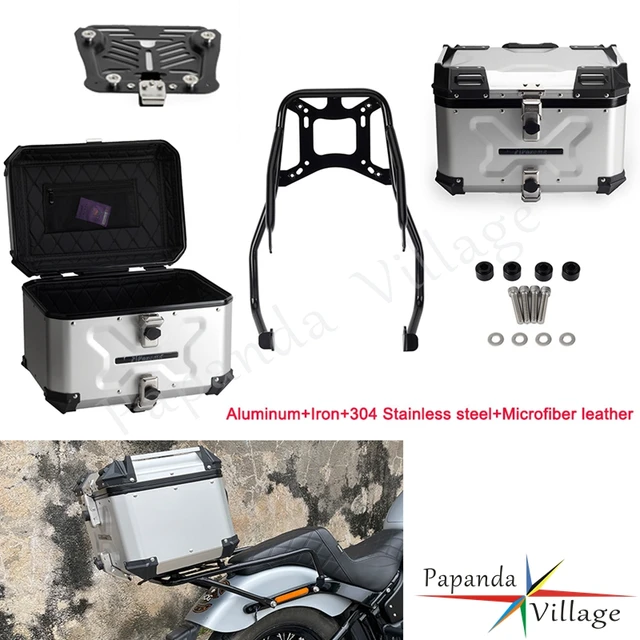This detailed series of photographs serves as an advertisement for a multifunctional storage box designed to be attached to the back of a motorcycle. The centerpiece of the images is a robust, silver box constructed from a combination of aluminum, iron, 304 stainless steel, and microfiber leather. The box features sleek black edges around the lid and is secured by a metal tube cage that supports its attachment to the motorcycle. One photo showcases the box in its closed state, while another reveals its entirely black interior when open. Accompanying images display the various screws and bolts necessary for installation, as well as the support frame or rack that secures the box to the bike. 

At the bottom left of the layout, a photograph illustrates the box mounted on a motorcycle, extending beyond the rear wheel. In the bottom right corner, the branding 'Papanda Village' appears in black letters, with a vibrant, angular star logo featuring green, red, yellow, and orange hues next to it. Centrally, between the motorcycle image and the parts of the storage box, red-pink text highlights the materials: "Aluminum + Iron + 304 Stainless Steel + Microfiber Leather." This comprehensive visual guide and branding emphasize the durability and design aesthetics of the motorcycle storage solution.